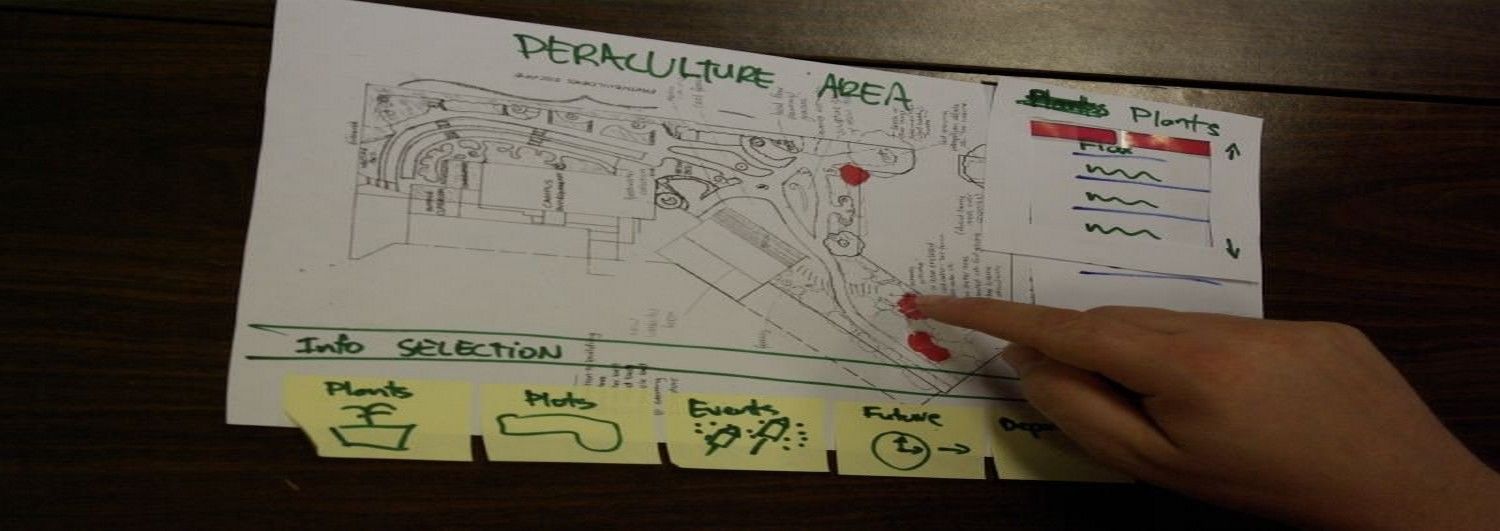In this indoor photograph, a Caucasian right hand extends from the lower right corner, its index finger pointing purposefully at a red dot on a white, rectangular piece of paper. The paper lays on what appears to be a dark brown, almost mahogany wooden surface, possibly a tabletop or floor, illuminated softly from the upper right. The paper features a simplistic hand-drawn map outlined in black ink with several lines and three notably red splotches. At the top of the paper, written in green marker, are the words "Permaculture Area." Below, on the left side, another green inscription reads "Info Selection." Adorning the bottom of the paper, small yellow sticky notes are attached, labeled in visible handwriting with words like "plants," "plots," "events," and "future," among others, partially obscured by the pointing hand. The overall arrangement evokes a sense of careful planning and organization, set against the rich, earthy tones of the wooden background.